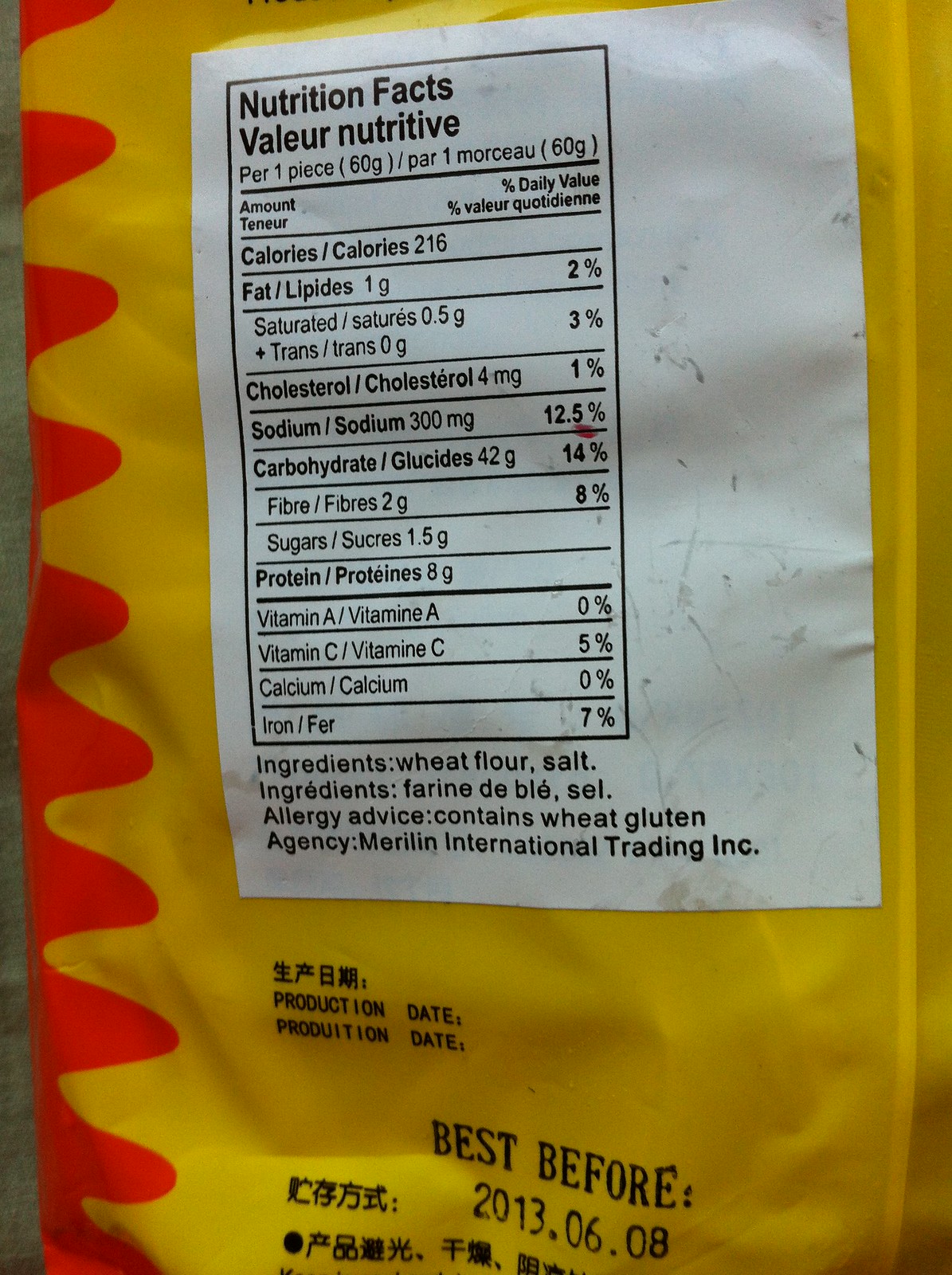This image features a nutritional facts label, predominantly in Chinese, indicating it belongs to a packaged food item. The "best before" date on the label is June 8, 2013. Despite the absence of an explicit production date, the term "production date" appears in Chinese characters.

At the top of the label, it states "Nutritional Facts per One Piece (60 grams)." The nutritional details are as follows:
- Calories: 216
- Total Fat: 1 gram
- Saturated Fat: 0.5 grams
- Trans Fat: 0 grams
- Cholesterol: 4 milligrams
- Sodium: 300 milligrams
- Total Carbohydrates: 42 grams
- Dietary Fiber: 2 grams
- Sugars: 1.5 grams
- Protein: 8 grams
- Vitamin A: 0%
- Vitamin C: 5%
- Calcium: 0%
- Iron: 7%

The ingredients listed include wheat flour and salt, suggesting that the product is likely a type of cracker. Allergy advice mentions that the product contains wheat gluten. The responsible entity is Maryland International Trading Incorporated. Additional text on the label appears to be in French.

The packaging is yellow with a distinctive wave of orange running down the left-hand side.